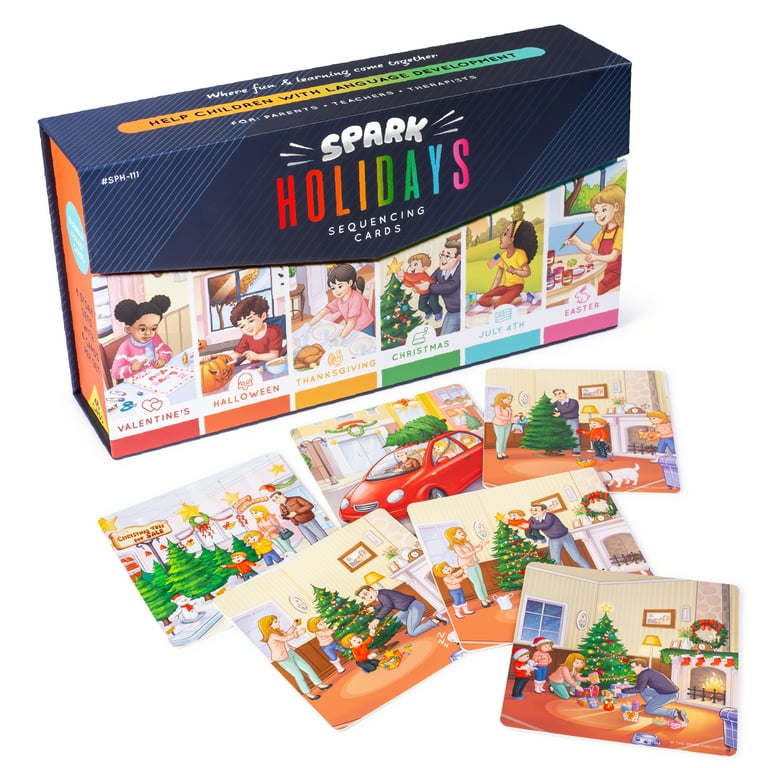The image features an advertisement-style photo of a box of "Spark Holidays Sequencing Cards" on a white background, taken from above. The top of the blue box displays the brand name "SPARK" in bold white letters, followed by "HOLIDAYS" in multi-colored text, and "SEQUENCING CARDS" below in smaller white letters. The top of the box also bears the slogan, "Where fun and learning come together. Help children with language development. For teachers, therapists, and parents."

The front of the box showcases six different holiday themes: Valentine's Day, Halloween, Thanksgiving, Christmas, July 4th, and Easter. Each holiday is illustrated with corresponding imagery featuring children engaged in relevant activities: an African-American girl making Valentine cards, a European descent boy carving a pumpkin for Halloween, a European descent girl painting with a Thanksgiving turkey, a father and son holding a Christmas tree, an African-American girl and her father with an American flag for July 4th, and a European descent girl painting Easter eggs.

In front of the box, six sequencing cards are displayed, all themed around Christmas. These cards depict various stages of the holiday: a child at the mall, shopping for a tree, driving the tree home with it secured on top of the car, setting up the tree, decorating it as a family, placing a star on the top, and finally showing presents under the fully decorated tree.